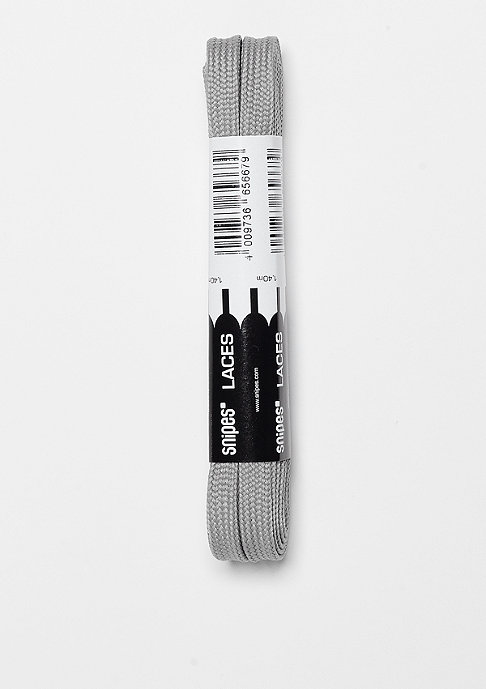The image is a straightforward monochrome photograph, taller than it is wide, featuring a close-up of a pair of thick, woven gray shoelaces wrapped tightly in their original store packaging. The shoelaces, likely intended for sneakers or running shoes, are centrally placed on an off-white background. The packaging consists of two parts: the top half displays a clear barcode with the product number on a white background, and the bottom half, on a black background, features the brand name "snipes" in lowercase and "LACES" in uppercase. The overall aesthetic of the image is minimalistic, focusing solely on the shoelaces and their packaging, with no additional elements in the composition.